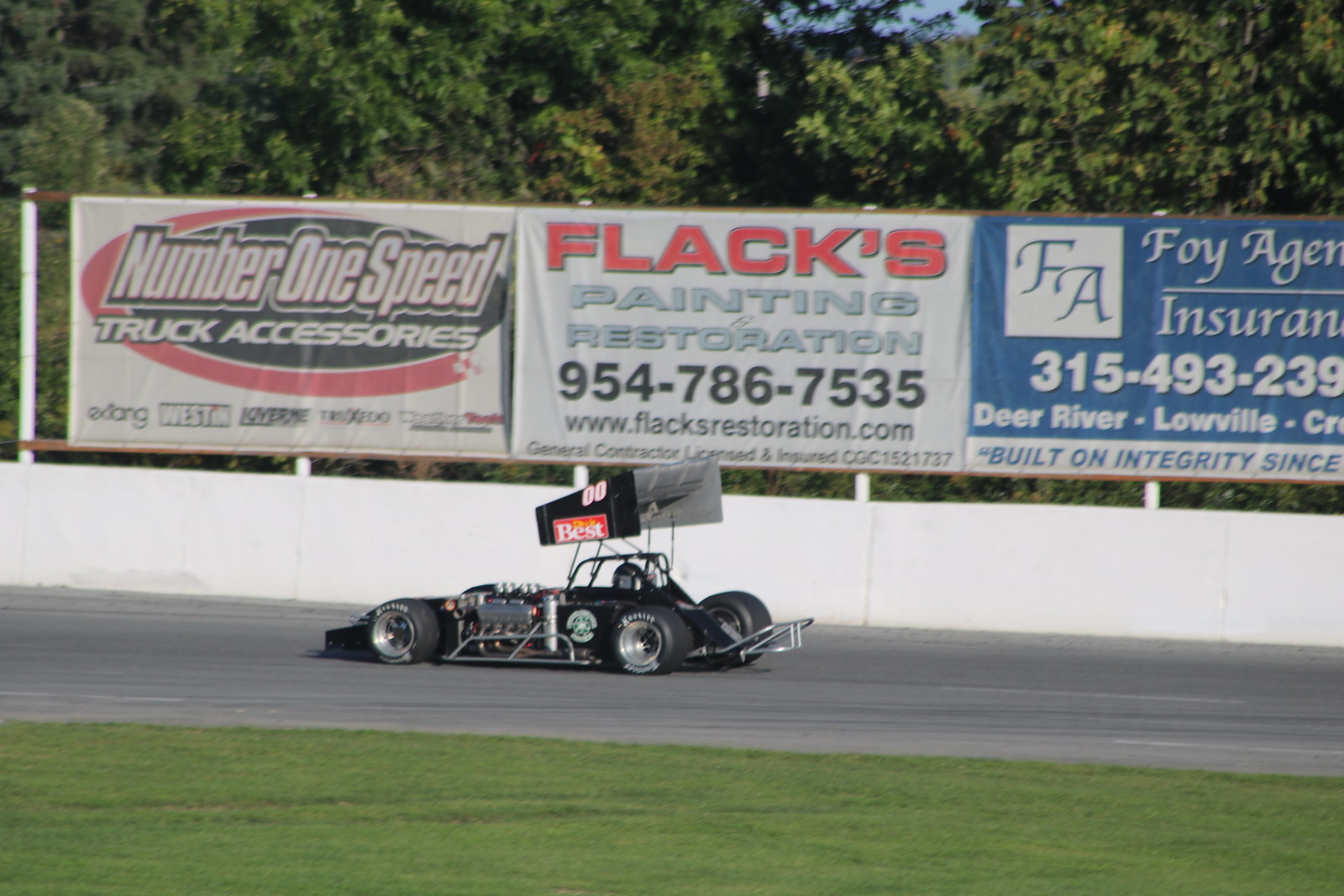The image depicts a scene at a racetrack. In the foreground, there is a vibrant patch of green grass leading up to a gray cement track. Dominating the center of the image is an open small race car, akin to a hot rod, featuring large, thick tires and a prominent white spoiler. The car itself is predominantly black and bears some decals or text, though they are not fully legible.

In the background, a white wall lines the side of the racetrack, adorned with several banners. The first banner promotes 'Number One Speed Truck Accessories.' Adjacent to it, the second banner advertises 'Flax Painting Restoration,' complete with a phone number and a website URL. The third banner, situated on the right, is blue and reads 'FOIA Agent Insurance,' though some of the text including a phone number and partial address information for locations such as Deer River and Lowville, is cut off.

Beyond the wall and banners, a cluster of trees is visible, adding to the outdoor setting. The top of the image shows a clear blue sky, indicating that this scene is illuminated by daylight. The overall composition, colors, and objects—from the grassy foreground to the detailed advertisements—suggest that this is a lively, bustling racetrack environment.